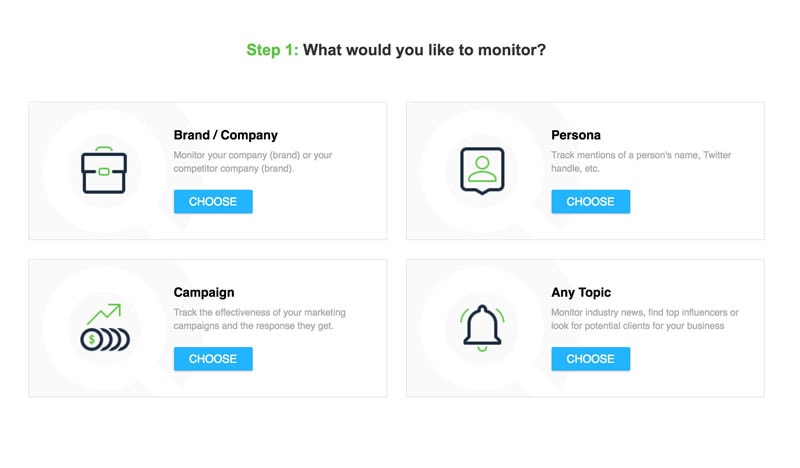The image displays a section of a website's interface focused on monitoring options. At the top of the page, "Step One: What would you like to monitor?" is prominently written in black text, prefaced by a green label.

The layout features a grid with four distinct sections:

1. **Top Left - Brand/Company:**
   - **Icon:** A small box with black lines.
   - **Description:** "Monitor your company (brand) or your competitor company (brand)" in black text.
   - **Button:** A blue "Choose" button.

2. **Top Right - Persona:**
   - **Icon:** A comic bubble with a green silhouette of a person.
   - **Description:** "Track mentions of a person's name, Twitter handle, etc." in black text.
   - **Button:** A blue "Choose" button.

3. **Bottom Left - Campaign:**
   - **Icon:** A stack of coins with a green upward arrow.
   - **Description:** "Track the effectiveness of your marketing campaigns and the response they get" in black text.
   - **Button:** A blue "Choose" button.

4. **Bottom Right - Any Topic:**
   - **Icon:** An alarm bell.
   - **Description:** "Monitor industry news, find top influencers, or look for potential clients for your business" in black text.
   - **Button:** A blue "Choose" button.

Each option is accompanied by a descriptive icon and a blue "Choose" button for selection, providing users with a clear and organized method to specify their monitoring preferences.